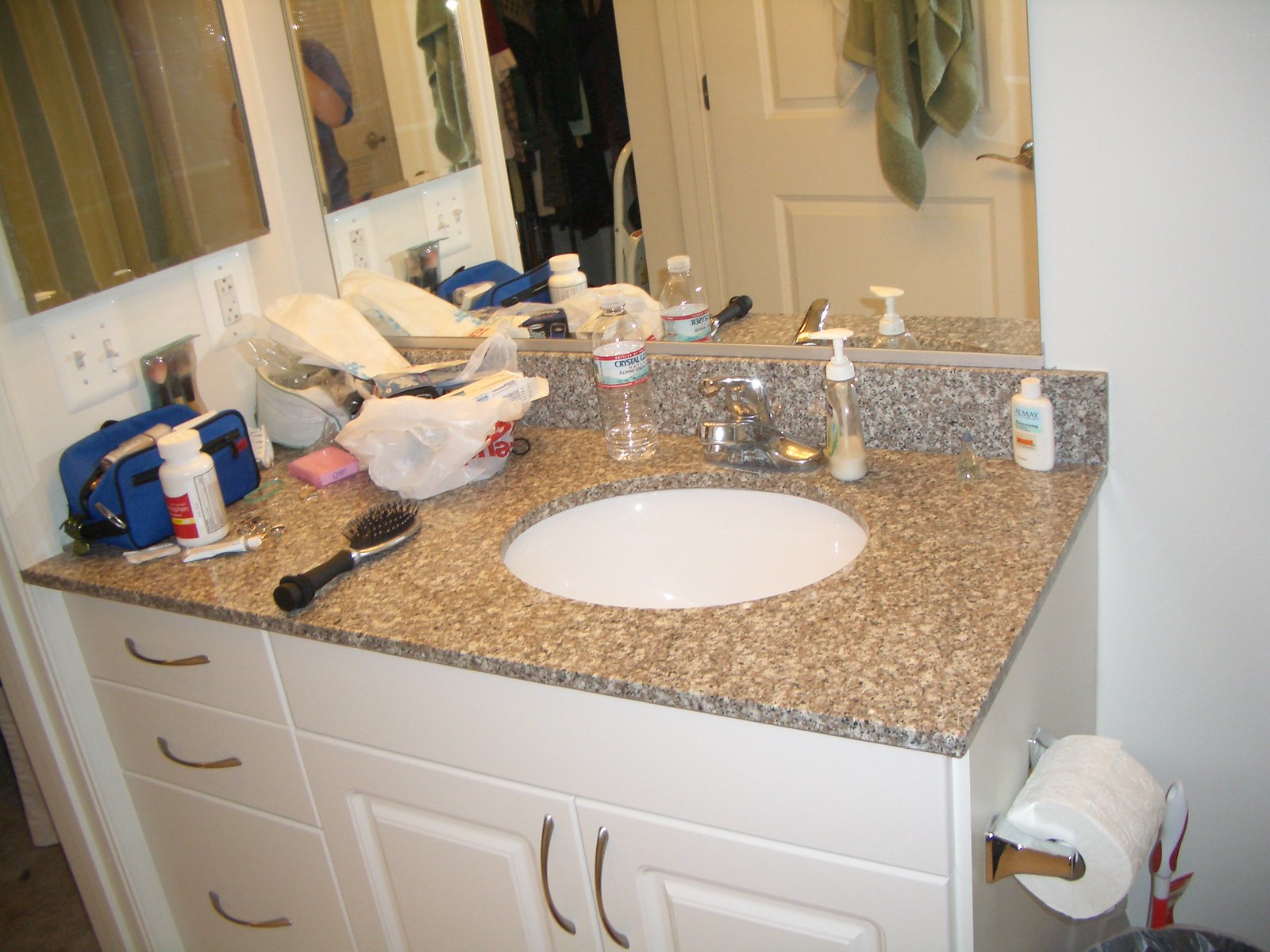This photograph captures a slightly underexposed bathroom vanity setup. The vanity features a white-front cabinet fitted with three drawers and two doors below the sink, each adorned with elegantly curved metal handles. The countertop boasts a granite-like surface with an under-mount white oval sink. A matching backsplash, approximately four inches tall, runs along the back but curiously not on the left side. 

The left wall, pristine white, extends down to the cabinet top and is equipped with a pair of classic toggle switches and an electrical outlet. Above these fixtures, there is a decorative element - possibly a wood pattern or a mirror reflecting part of the shower. 

A large mirror sits above the countertop, reflecting a door that appears to be ajar, with a green towel hanging from it, and the doorway visible further to the left. Scattered across the countertop are several tubes of hand lotion, adding a lived-in touch to the scene.